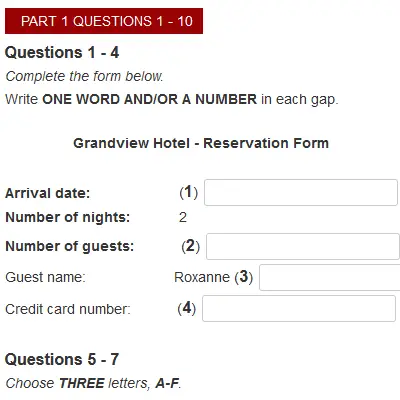The image displays a section of a form with detailed instructions in both text and graphic elements. At the top, there's a horizontal maroon bar, not quite bright red, with the text "Part 1: Questions 1 through 10" written in white letters. Beneath this heading, the text for questions 1 through 4 appears in black font, which reads: "Complete the form below. State one word and/or a number in each gap."

Below this instruction, the form is titled "Grandview Hotel Reservation Form." The form fields are as follows:
- Arrival date: [Blank]
- Number of nights: 2
- Number of guests: 2
- Guest name: Roxanne
- Credit card number: [Blank] 

Notably, the answers to "Arrival date," "Number of guests," "Guest name," and "Credit card number" appear next to the respective fields within parentheses but are not inside the fields themselves.

For questions 5 through 7, the instruction reads: "Choose" with the word "three" emphasized in all bold letters, followed by options labeled A through F. The form fields and instructions are clearly delineated, though the exact answers within the parantheses suggest they may not be final or properly placed.

Overall, the image depicts a partially completed hotel reservation form with clear instructions for filling out the remaining fields.